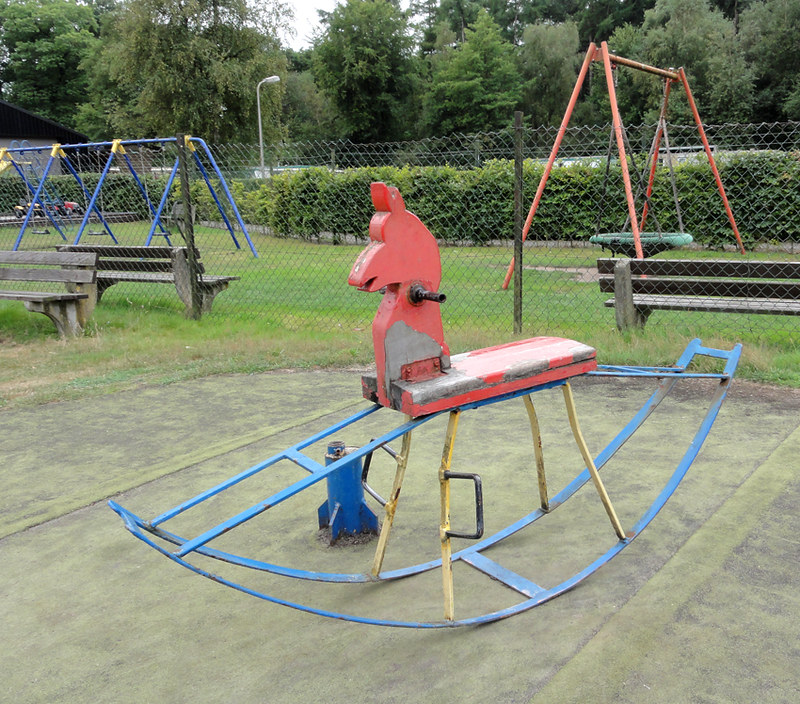A detailed photograph captures an empty neighborhood playground. In the forefront, there's a distinctive red metal rocking toy shaped like a seahorse or llama, equipped with a hat, two handles, and footrests. The rocking toy sits on four yellow legs attached to curved metal bases, allowing it to rock back and forth. This toy is positioned on a flat, slightly weathered concrete surface that was likely part of an old parking lot, now overlaid partially with grass.

The playground area is enclosed by a chain-link fence, beyond which lush green trees and bushes can be seen. Towards the left, there is a blue metal swing set with four bars that likely supported multiple swings, but only a large, bowl-shaped swing seat remains visible. Additional wooden benches are scattered along the perimeter outside the fence, adding to the communal feel of the space.

Above the scene, the sky is mostly white, creating a stark contrast with the vibrant colors of the playground equipment and greenery. The serene atmosphere, combined with the absence of people, suggests an inviting but underutilized community space.